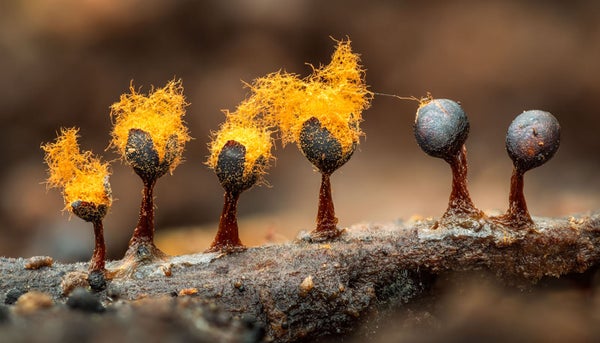The photograph showcases a close-up of seven distinctive mushrooms arranged in a row on a gray, bare, and rocky ground. Each mushroom features a round black head atop a brown stalk. Notably, the four mushrooms on the left side are adorned with a large mass of yellow, fuzzy, spore-like substances emerging from their tops, resembling lines or fur. Conversely, the two mushrooms on the right side appear undisturbed, showing no such substances, except for a yellow line connecting the middle mushroom to the top of the second right mushroom. The background is blurred, showing only indistinguishable dark and light brown hues, likely indicating a natural outdoor setting.